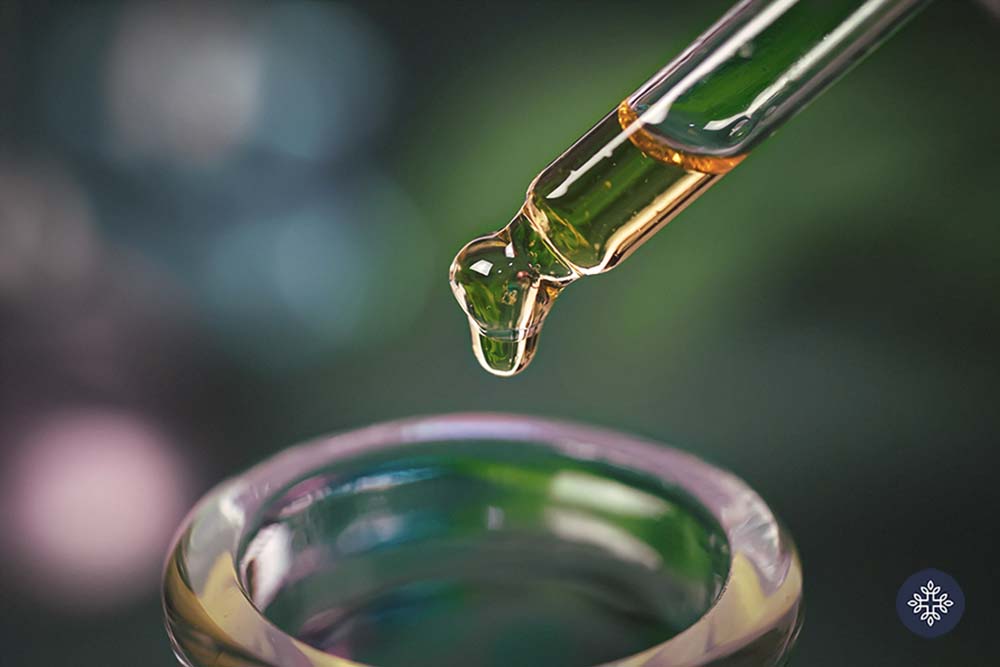The image is a close-up of a precise chemistry experiment, capturing a thick, amber-tinted liquid being carefully dropped from a small, glass dropper with a short, rounded tip into a clear, glass bowl. The dropper is positioned at the top right, directing the liquid towards the center of the image. The background is a blurred mosaic of greens, pinks, and blues, making it impossible to discern any specific objects, though some small lights are visible to the left. In the lower right-hand corner, there's a blue symbol resembling a plus sign surrounded by leaf-like designs, possibly indicating a connection to chemistry or medicine. The overall focus is on the meticulousness of the liquid being dropped, ensuring precise measurement.